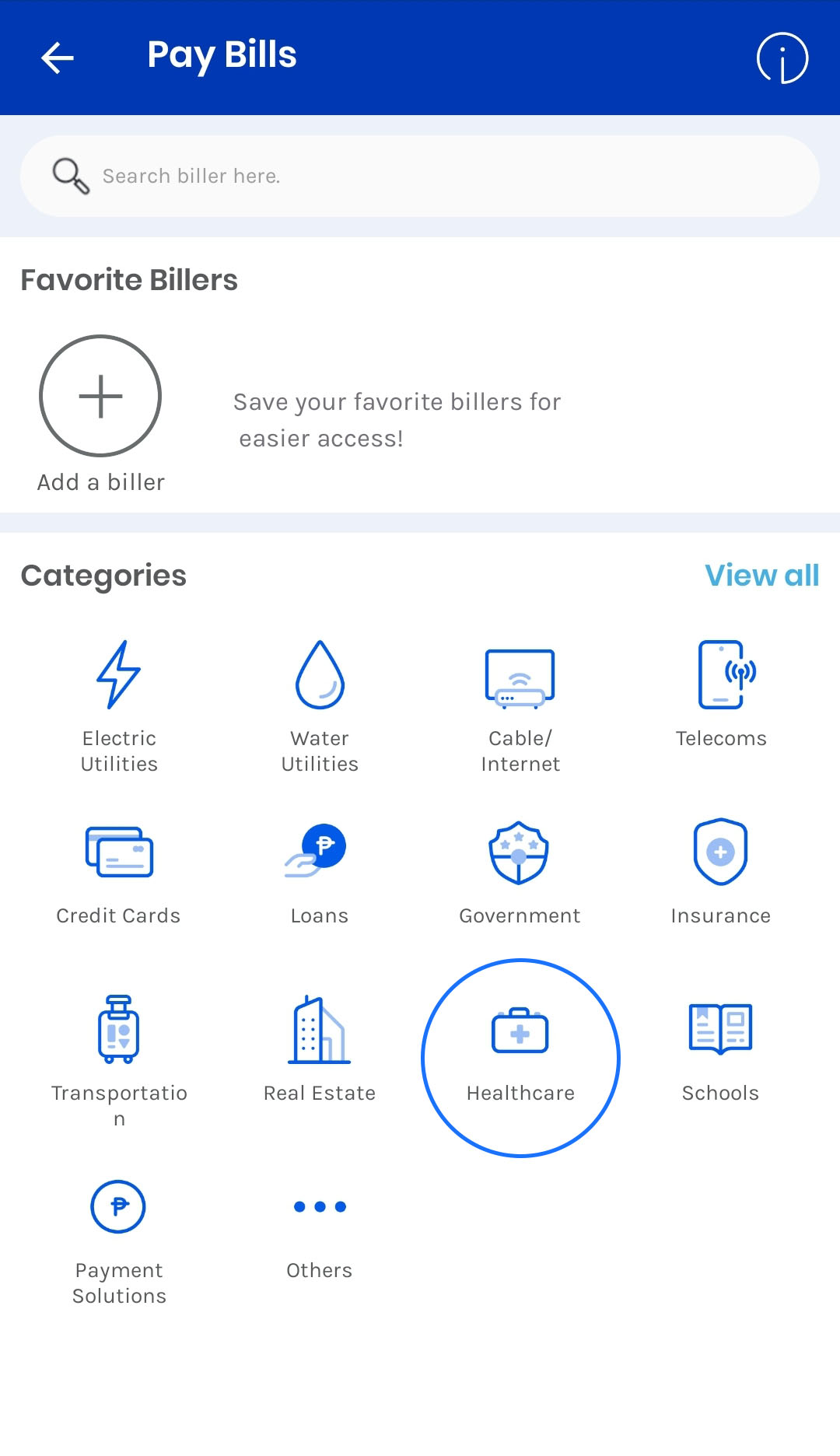This screenshot displays a mobile application's interface for managing bill payments. At the top left corner, there is a back arrow icon, followed by the title "Pay Bills" highlighted in a blue banner. On the right side of this banner, there's an information icon, represented by a white circle with an 'i' inside it.

Beneath the banner, a search field adorned with a magnifying glass icon invites users to "Search biller here." Below this search bar, the section "Favorite Billers" is displayed, accompanied by a circle with a plus sign to add favorite billers. Adjacent to the plus sign, a message reads, "Save your favorite biller for easier access!"

The next section, labeled "Categories," is positioned under the "Favorite Billers" heading and features a "View All" option in blue font on the right. This section showcases 14 categories of billers, arranged in a grid layout with four across in the first row, three in the second row, and two in the third row. The categories listed are as follows:

1. Electric Utilities – Icon: Lightning Bolt
2. Water Utilities – Icon: Water Drop
3. Cable Internet – Icon: TV with a Router and Wi-Fi signal
4. Telecoms – Icon: Smartphone
5. Credit Cards – Icon: Credit Cards
6. Loans – Icon: Generic Loan Symbol
7. Government – Icon: Shield
8. Insurance – Icon: Shield with a Plus Sign
9. Transportation – Icon: Transportation-Related Symbol
10. Real Estate – Icon: Simple Buildings
11. Healthcare – Icon: First Aid Kit with a Medical Cross (Circled in Blue)
12. Schools – Icon: School-Related Symbol
13. Payment Solutions – Icon: Payment-Related Symbol
14. Other – Icon: Miscellaneous Symbol

All icons are uniformly designed in blue, ensuring a consistent look across the interface. The rest of the screen below these icons is white.